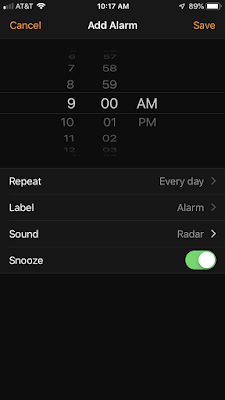Screenshot of a smartphone displaying the alarm setup page within what appears to be the clock application. At the top left of the screen, the carrier "AT&T" is visible, confirming the device is connected to their network. The current time is shown in the center at "10:17 AM," and the battery indicator at the top right reveals a charge level of 89%.

In the alarm setup interface, the header reads "Add Alarm" in white text. On the top left, there's an orange "Cancel" button, while an orange "Save" button is situated on the top right, allowing the user to finalize or discard their changes. 

In the central part of the screen, a time picker displays the alarm set for "9:00 AM." Underneath the time picker, several customizable options are listed:

- **Repeat:** Set to "Every day," indicating that the alarm will recur daily at 9:00 AM.
- **Label:** Named "Alarm," potentially for organizational purposes or for a specific task.
- **Sound:** Set to "Radar," determining the audio tone that will play when the alarm goes off.
- **Snooze:** Toggled on, giving the user the option to snooze the alarm when it activates.

These settings suggest a carefully configured daily wake-up alarm designed for consistency and customizable functionality.